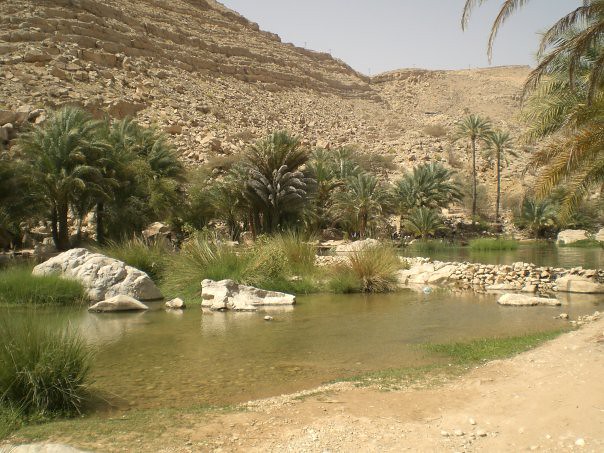This photograph, taken on an overcast day, captures a serene outdoor scene featuring a small, shallow body of water, likely a pond. In the distance on the right side, there is more water and some dry land composed of brown sand and little stones. The water appears murky and has algae where it meets the shore. Dotting the water and the middle section are large, sun-bleached rocks, through which some grass is growing. Toward the right-hand side, there is also a small rock wall. In the background, rows of trees with spiky leaves can be seen, with an imposing dirt hill or mountain towering even further back. The sky is visible above, completing this tranquil natural setting.